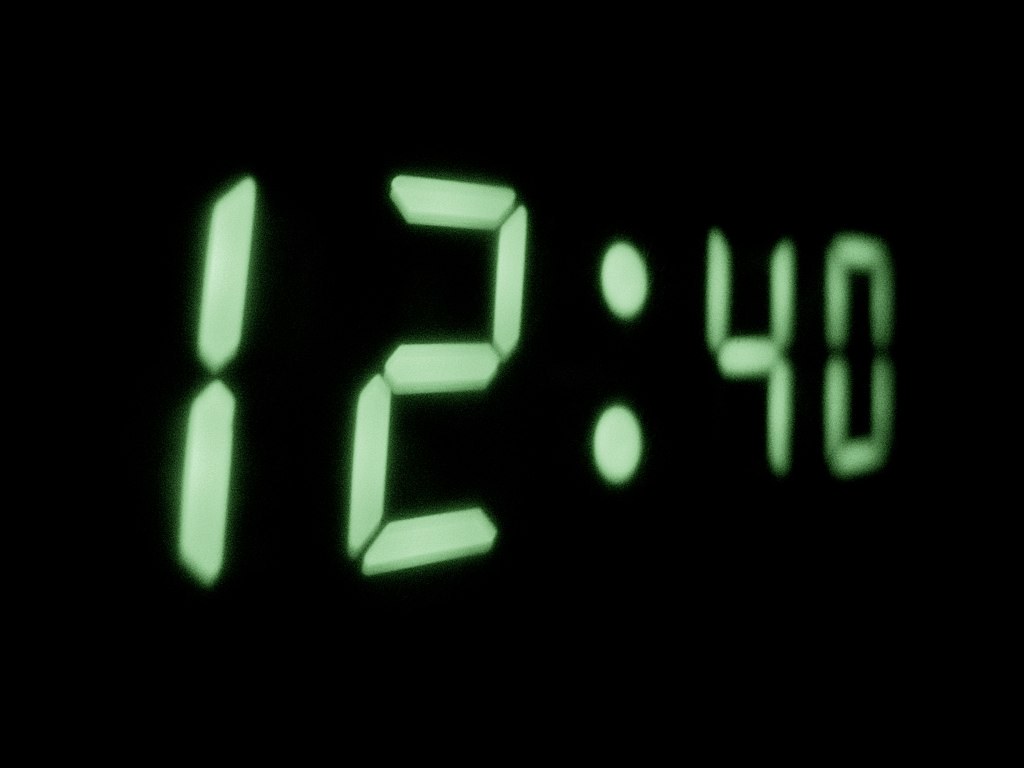This photograph captures a close-up of a digital clock face, prominently displaying the time "12:40" in luminous green numerals. The image is predominantly enveloped in darkness, emphasizing the glowing digits. The clock is angled slightly from the left, causing a light blur on the first digit of "12" and the last digit of "40." The scene suggests the clock is likely an alarm clock in a dimly lit room, with no other visible elements to distract from the focus on the time.